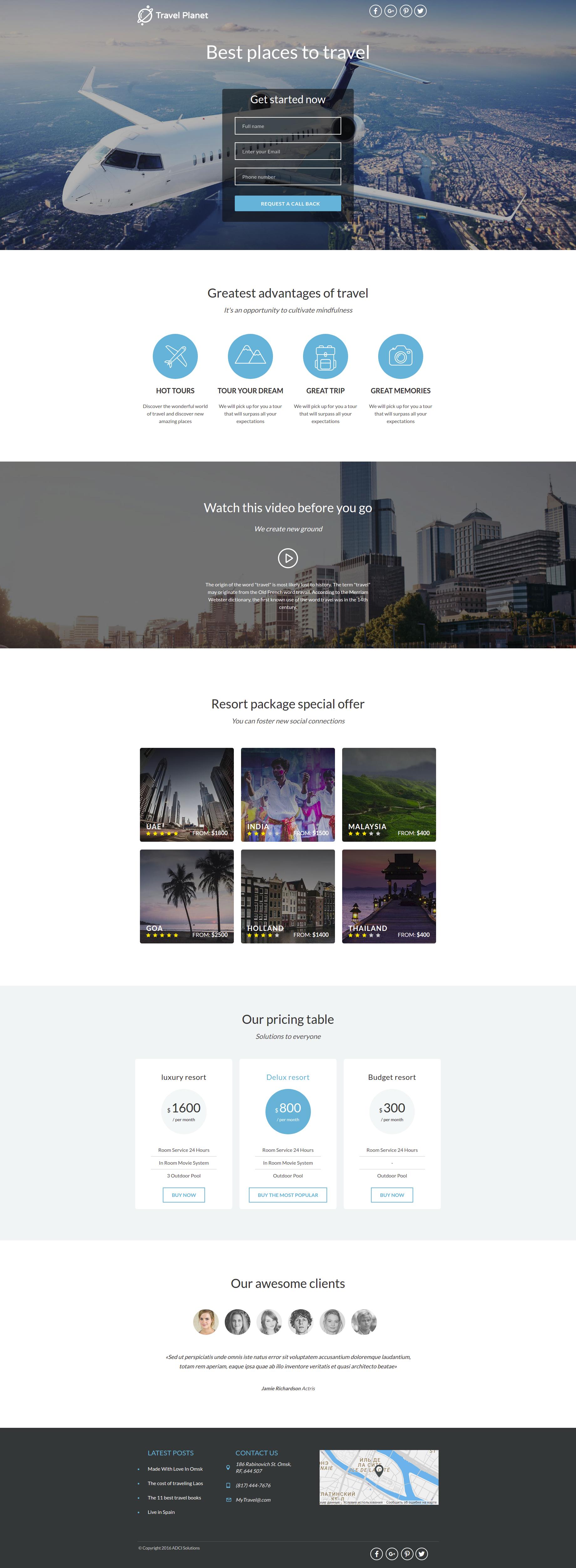### Website Overview: Travel Planet

#### Header Section
- **Header:** The top header displays the brand name "Travel Planet" on the upper left.
- **Social Media Icons:** In the upper right are circular icons for Facebook, Google+, Pinterest, and Twitter. 

#### Hero Section
- **Hero Image Text:** Centered on the hero image is the phrase "Best Places to Travel" in white text.
- **Vertical Form:** Below this text is a translucent black form labeled "Get Started Now" in white.
  - **Form Inputs:** 
    - Full Name
    - Enter Your Email
    - Phone Number
  - **Submit Button:** Labeled "Request a Call Back."

#### Advantages of Travel Section
- **Main Heading:** "Greatest Advantages of Travel"
- **Subheading:** In italics, it says, "It's an opportunity to cultivate mindfulness."
- **Background:** White

#### Features Section
- **Feature 1: Hot Tours**
  - **Icon:** Blue icon with a plane
  - **Description:** "Discover the wonderful world of travel and amazing new places."

- **Feature 2: Tour Your Dream**
  - **Icon:** Blue circle with a mountain
  - **Description:** "We will pick up a tour for you that will surpass all your expectations." *(Note: The phrase includes grammatical errors.)*

- **Feature 3: Great Trip**
  - **Icon:** Blue icon with a book bag outline
  - **Description:** "We will pick up a tour for you that will surpass all your expectations." *(Repeated grammatical error.)*

- **Feature 4: Great Memories**
  - **Icon:** Blue and white icon with a camera outline
  - **Description:** "We will pick up a tour for you that will surpass all your expectations." *(Repeated grammatical error.)*

#### Video Section
- **Heading:** "Watch This Video Before You Go"
- **Description:** "We create new ground" with a play button icon (circle with a triangle) suggesting a video.

#### Special Offers
- **Heading:** "Resort Package Special Offer"
- **Pricing Table:**
  - **Luxury Resort:** $1,600 per month (Includes 24-hour room service, in-room movie system)
  - **Deluxe Resort:** $800 per month
  - **Budget Resort:** $300 per month

#### Clients and Location
- **Heading:** "Our Awesome Clients"
- **Ending Section:** Displays a map showing the location.

This website offers a structured and appealing layout filled with essential travel information, although some grammatical refinements are needed for a more professional presentation.